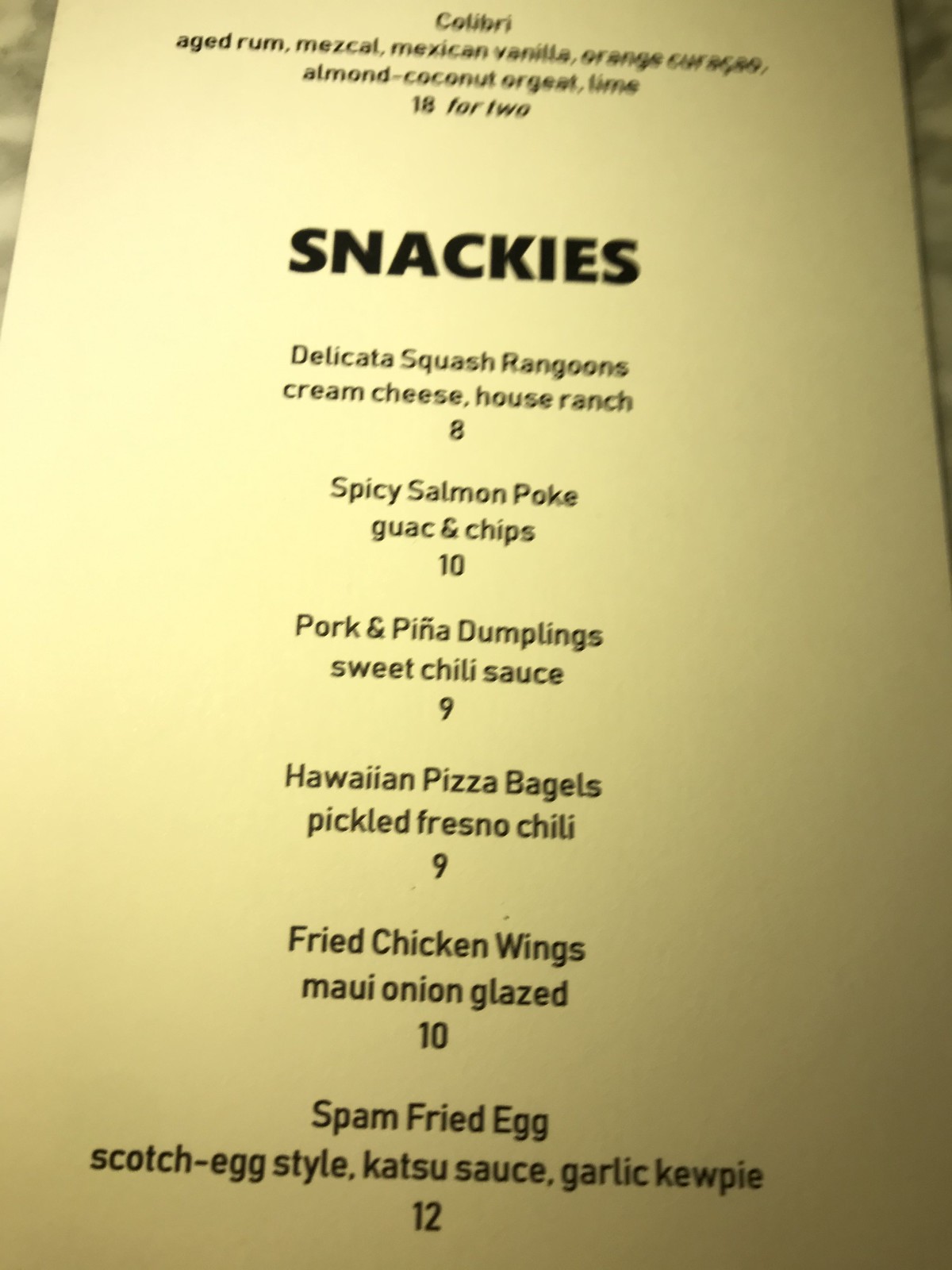A section of a high-class menu is displayed on a creamy white card. The top part is slightly cut off, but the word "Colibri" is visible, indicating a drink composed of aged rum, mezcal, Mexican vanilla, orange curacao, almond, coconut, or yet another ingredient (possibly a typographical error or a unique ingredient), and lime, priced at $18, with an additional note in italics specifying that the price is for two.

Below, in bold, the heading "Snackies" introduces a list of gourmet snacks:

- Delicata Squash Rangoons: Stuffed with cream cheese and served with house ranch dressing, priced at $8.
- Spicy Salmon Poke: Accompanied by guac and chips, for $10.
- Pork and Peanut Dumplings: Served with a sweet chili sauce, priced at $9.
- Hawaiian Pizza Bagels: Topped with pickled Fresno chili, for $9.
- Fried Chicken Wings: Glazed with Maui onion, available for $10.
- Spam Fried Egg, Scotch Egg Style: Paired with katsu sauce and garlic kuppi (a type of garlic-enhanced Japanese mayonnaise), priced at $12.